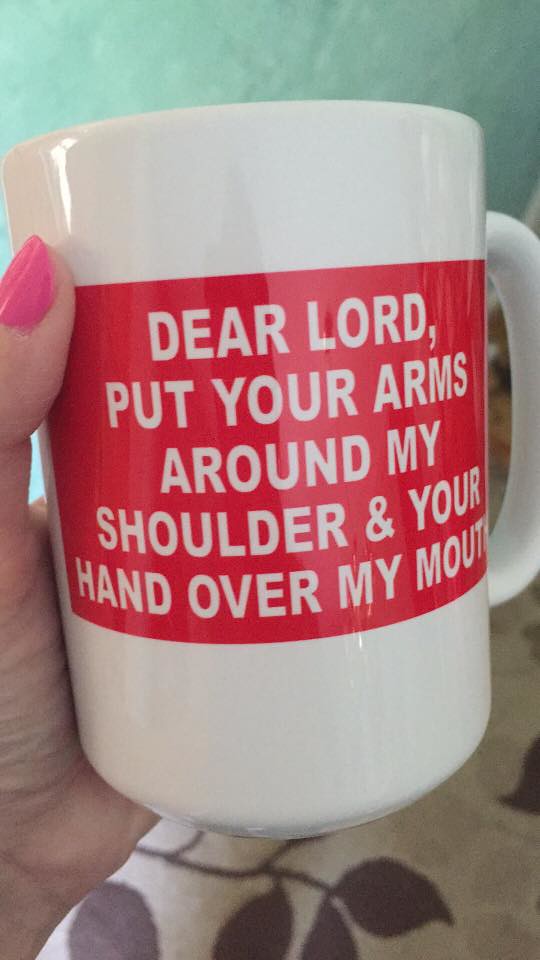The image features a white mug being held by a woman's left hand, recognizable by the pink nail polish on her thumbnail. The mug has a prominent red rectangular area with a humorous yet prayerful message in uppercase white letters: "DEAR LORD, PUT YOUR ARMS AROUND MY SHOULDERS AND YOUR HAND OVER MY MOUTH." In the background, a light green textured wall is visible, and below the mug is a surface that appears to be a carpet or tablecloth adorned with purple flowers or leafy vines. The scene reflects off the shiny mug surface, hinting at a possible doorway behind the person holding it.